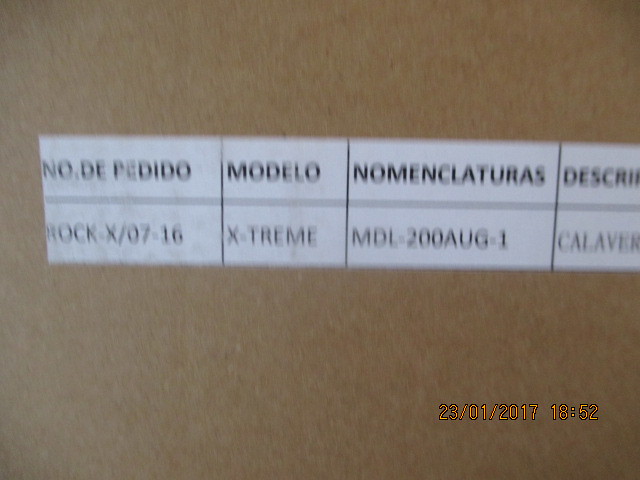The image displays a slim, rectangular white chart with four visible columns and two rows. The far-right column is partially cut off. The headers in the top row from left to right are labeled as follows: "NO. DE PEDIDO," "Modelo," "Nomenclaturas," and a cutoff "Descri." In the first row beneath these headers, the entries read: "ROCK-X-07-16," "X-TREME," "MDL-200AUG-1," and a partially visible "CALAVER." Additionally, in the bottom right-hand corner of the chart, a timestamp reads "23-01-2017 18:52."